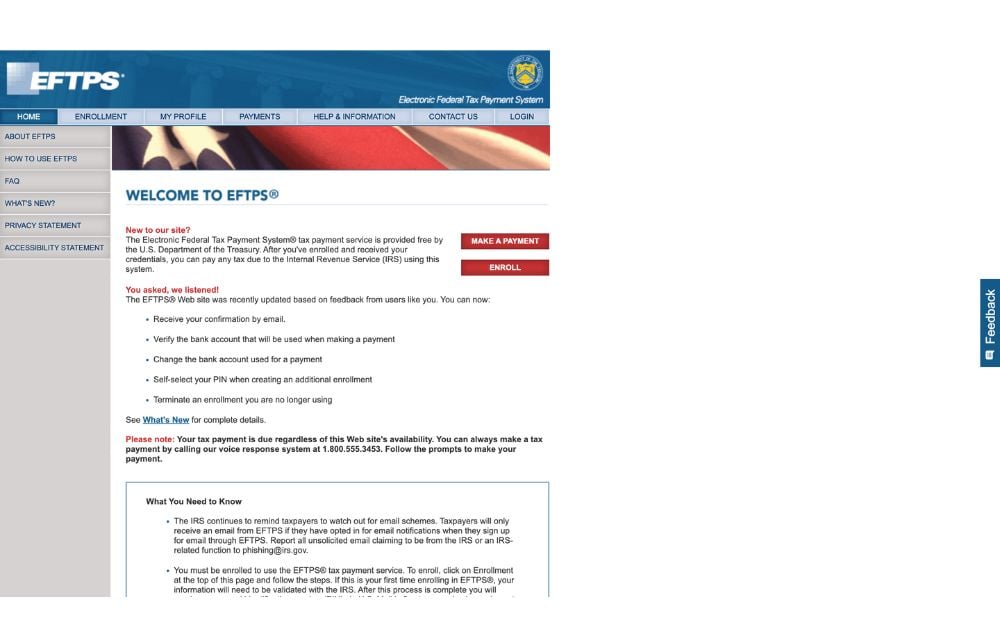Screenshot of a Website

The screenshot is rectangular, with longer left and right sides compared to the top and bottom edges. At the very top of the website, there is a prominent blue banner. In the top left corner of this banner, a gradient white square shifts from whiter at the top left to more gray at the bottom right. Slightly overlapping this gradient and positioned to its right is the website's name, rendered in large, bold, white capital letters: E-F-T-P-S. In the top right corner of the blue banner, there is a shield logo, and below it, white text reads: "Electronic Federal Tax Payment System."

Just below the blue banner are multiple clickable options for the user, aligned horizontally. The leftmost option is a blue rectangle with white text that says "Home." The remaining options are gray rectangles with blue text, listed from left to right as: "Enrollment," "My Profile," "Payments," "Help Information," "Contact Us," and "Login."

On the left side of the page, there are various other clickable options displayed as gray rectangles with blue text on a gray background. From top to bottom, these options read: "About E-F-T-P-S," "How to Use E-F-T-P-S," "FAQ," "What's New," "Privacy Statement," and "Accessibility Statement."

The main body of the website features a combination of black and red text set against a white background. The text content includes key information pertinent to the Electronic Federal Tax Payment System, providing users with detailed guidance and instructions.